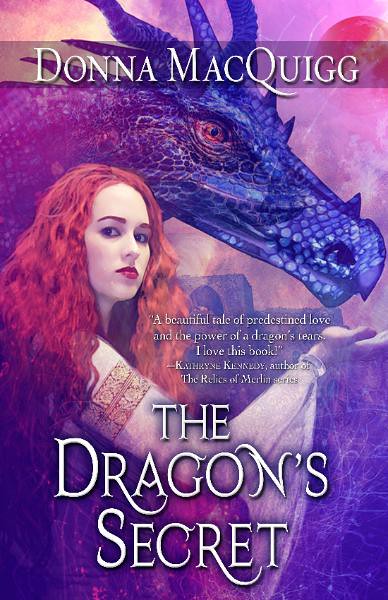The book cover for "The Dragon's Secret" by Donna McQuigg features an ethereal scene dominated by a woman and a dragon. The woman has long, flowing red hair, parted in the center, with slightly wavy locks cascading down. Her pale white skin is accentuated by her sheer, ancient-style dress, which drapes down to her wrists. She stands in a profile position, her body facing right while she turns her head towards the viewer with an intense gaze. Her arms are extended out and upwards as if poised to cup or hold something near her. 

In the background, a striking dragon emerges with blue and black scales that fade into purple hues. It boasts fierce red eyes and prominent horns. The dragon's head is positioned near the woman’s hands, giving a sense of interaction between them. Behind this pair, the backdrop is awash in a mystical blend of purple, pink, and red light, reminiscent of fire or the vibrant hues of a sunset filtering through clouds.

The cover text is both bold and delicate, with the author’s name, Donna McQuigg, prominently displayed at the top in large white letters. Near the woman’s extended arms, smaller white text reads: “A beautiful tale of predestined love and the power of a dragon's tears.” Below, the text credits this quote to Catherine Kennedy, author of “The Relics of Merlin's Service.” Finally, at the bottom of the cover, in large bold white letters, the title "The Dragon's Secret" stands out, anchoring the composition.